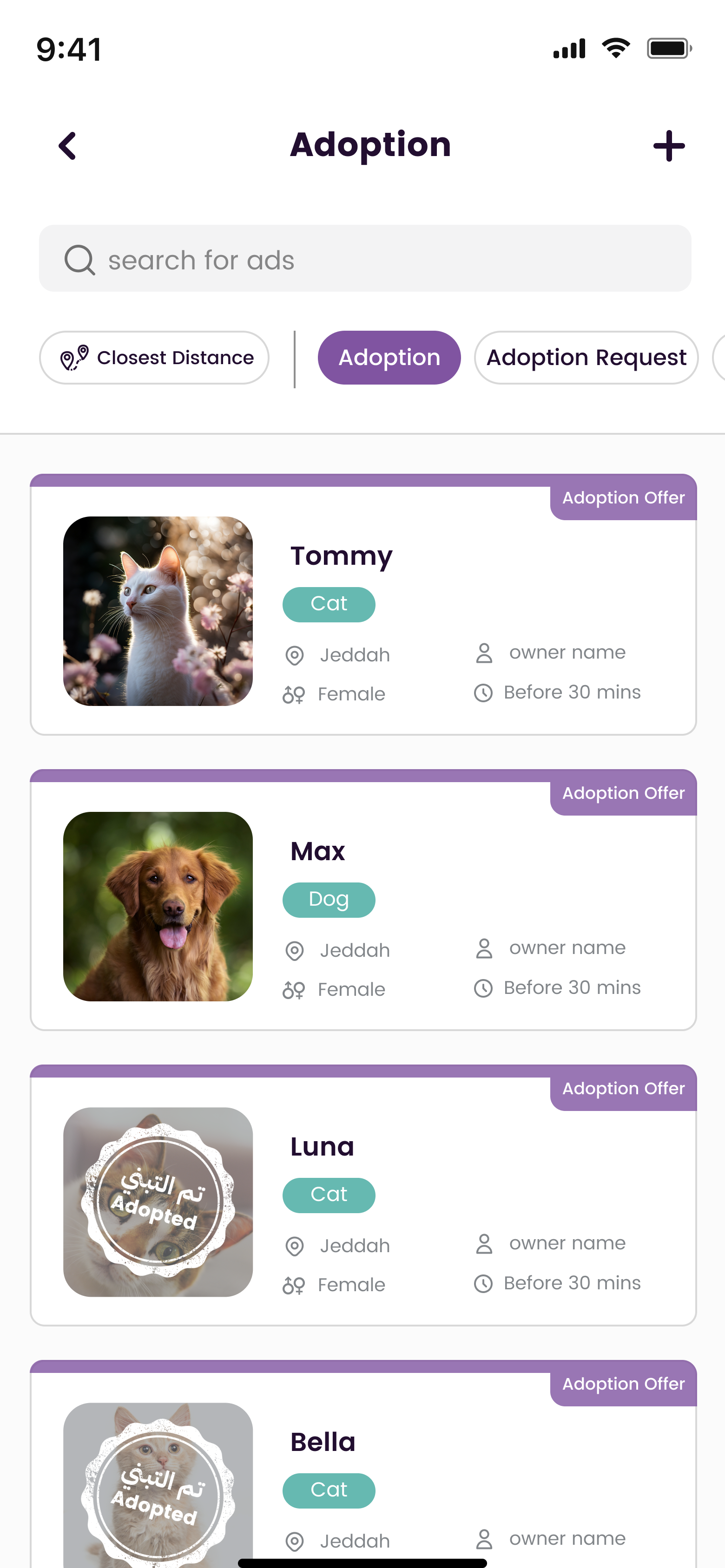This is an adoption page from an animal society featuring various pets available for adoption. The webpage allows users to sort animals by closest distance using designated buttons. A prominent purple button marked "Adoption" provides access to adoption information and procedures. The page showcases several animals with their respective images and details. 

Highlighted on the page is Tommy, a white cat pictured sitting amidst a bed of pink flowers. Beside Tommy's photo are details including gender, marked as female, and location, noted as Jeddah. The owner's name is listed, and there is a perplexing note "before 30 minutes," the meaning of which is unclear.

Another featured pet is Max, a golden retriever type dog. To the right of the main animal images is a section for adoption requests, where users can request more information about any of the animals displayed if they are interested.